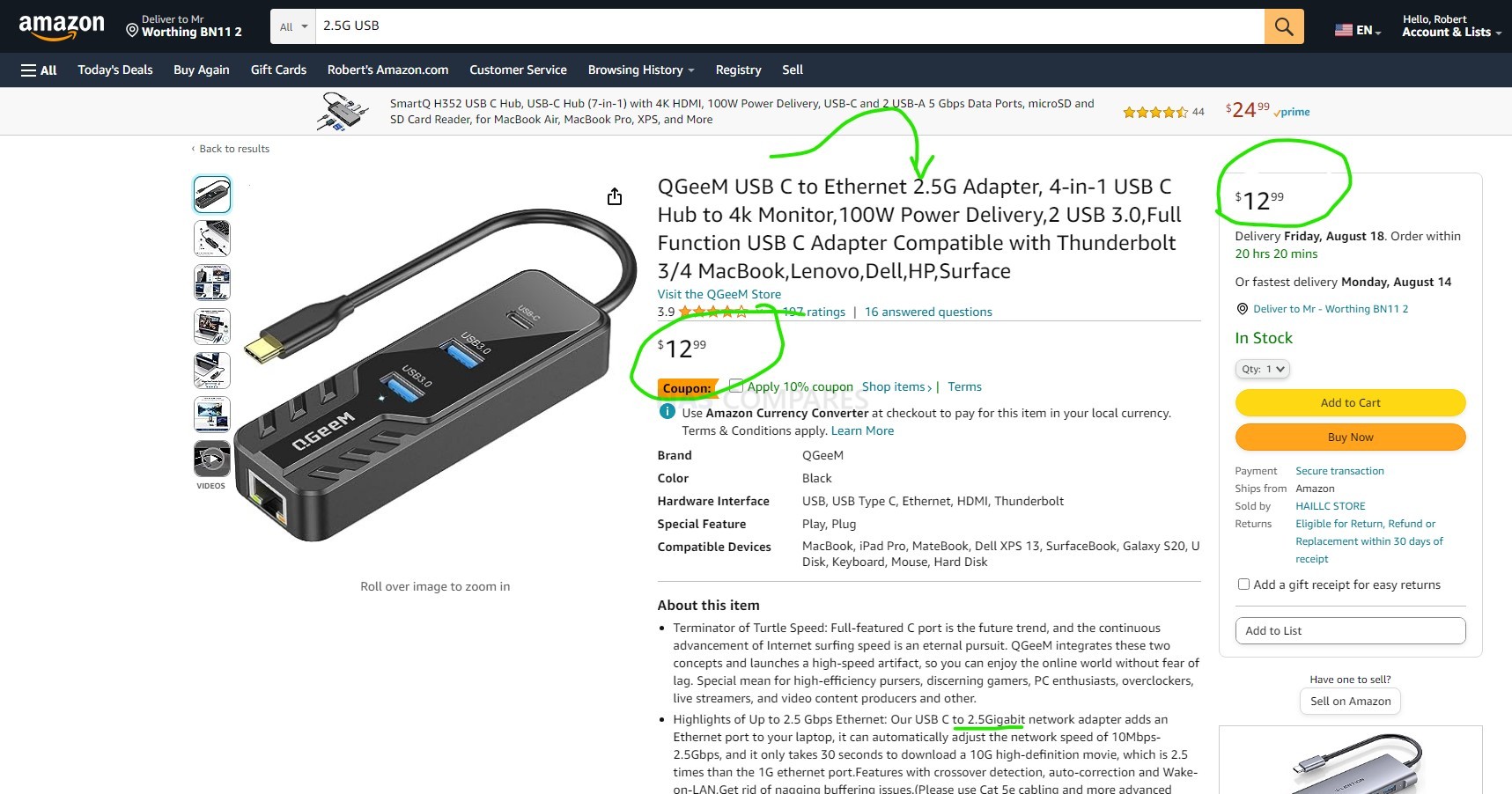**Detailed Caption:**

The screenshot captures an Amazon webpage with a predominantly black header. On the left side of the header, the iconic Amazon logo is displayed—featuring the trademark arrow swooping from 'A' to 'Z' in orange. Adjacent to the logo, the phrase "Delivering to" followed by the recipient's details is shown. The central search bar is white, with the search query "2.5G USB" entered into it. On the right side of the header, options to change the language to English and access the user's account, indicated as "Hello, Robert," are visible.

Beneath the header, on a grayish background with black and white text, several navigational links are listed, including "All of Today's Deals," "Buy Again," "Gift Orders," "Customer Service," "Browsing History," "Registry," and "Sell."

The main section of the screenshot, set against a white background, features a product listing for a black USB to Ethernet adapter. The device is plugged in, displaying an Ethernet port on its left side. The product name reads "QGM USB to Ethernet 2.5G Adapter." Annotations include an arrow pointing to the "2.5G" specification and the price, listed in red as $12.99, circled in green. Additionally, a 10% off coupon is indicated, also circled in green, highlighting a good deal for this 2.5 gigabit Ethernet adapter.

Someone has presumably drawn these annotations to emphasize the significant details and the deal, suggesting that they are securing a useful 2.5 gig adapter for their computer.

---
The caption you've requested is very descriptive, incorporating all aspects mentioned in your initial transcription while targeting an audience familiar with navigating e-commerce platforms. If you need it tailored differently, such as for a specific purpose or audience, please let me know!